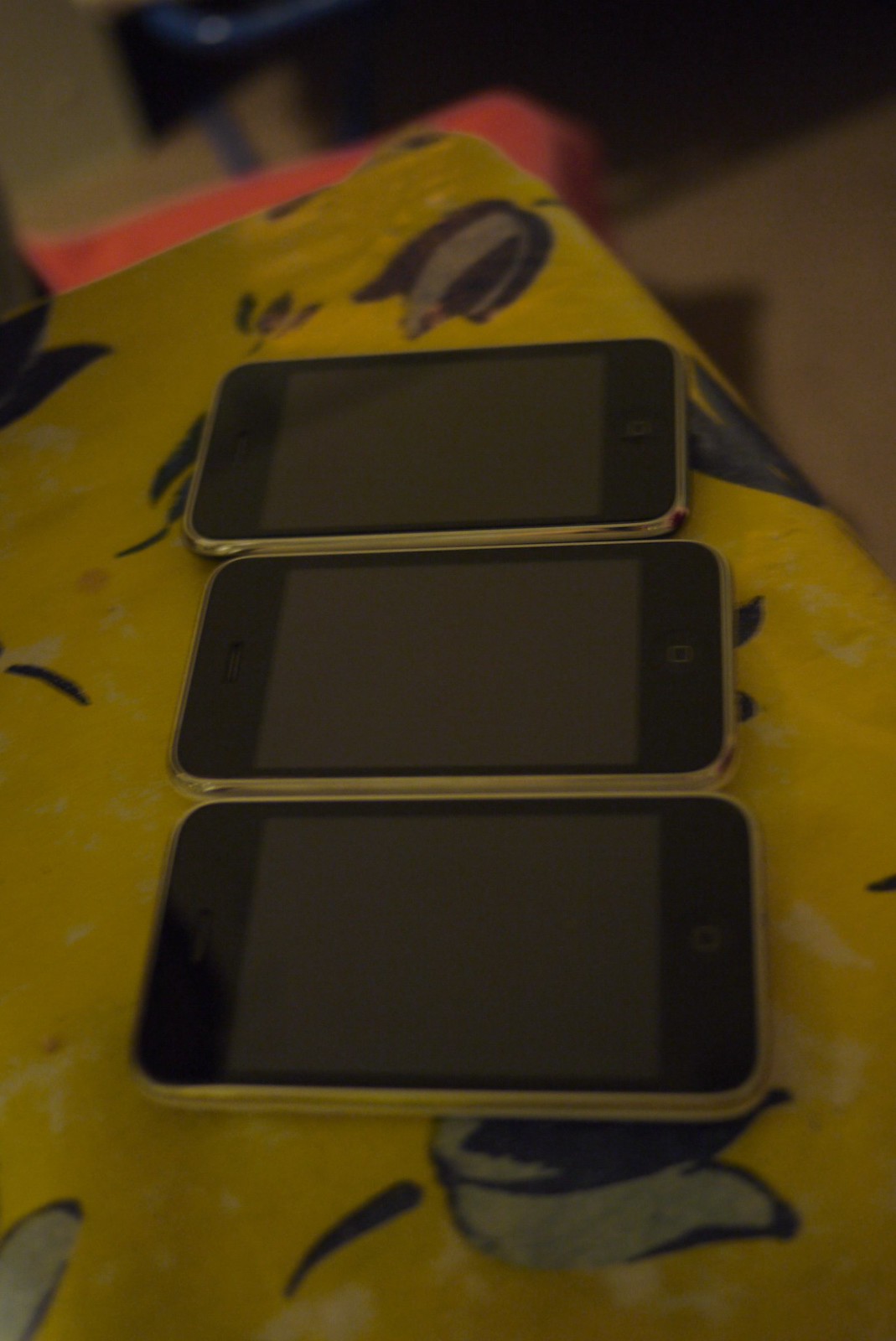The image depicts three identical, extremely old-style iPhones arranged in a slightly offset stack atop a yellow tablecloth adorned with a dark blue and light blue floral pattern, featuring black tulip or floral designs. Each iPhone has a silver outer rim, a black screen with a singular button on one end, a speaker on the other, and a small rectangular-shaped screen in the middle. The phones are turned off and show no display. The tablecloth appears to be plastic, and the photo is taken from a slightly overhead high angle, resulting in a somewhat blurry and out-of-focus image. In the far background, a light beige carpet or floor is visible along with a red fabric or object, possibly part of a chair.